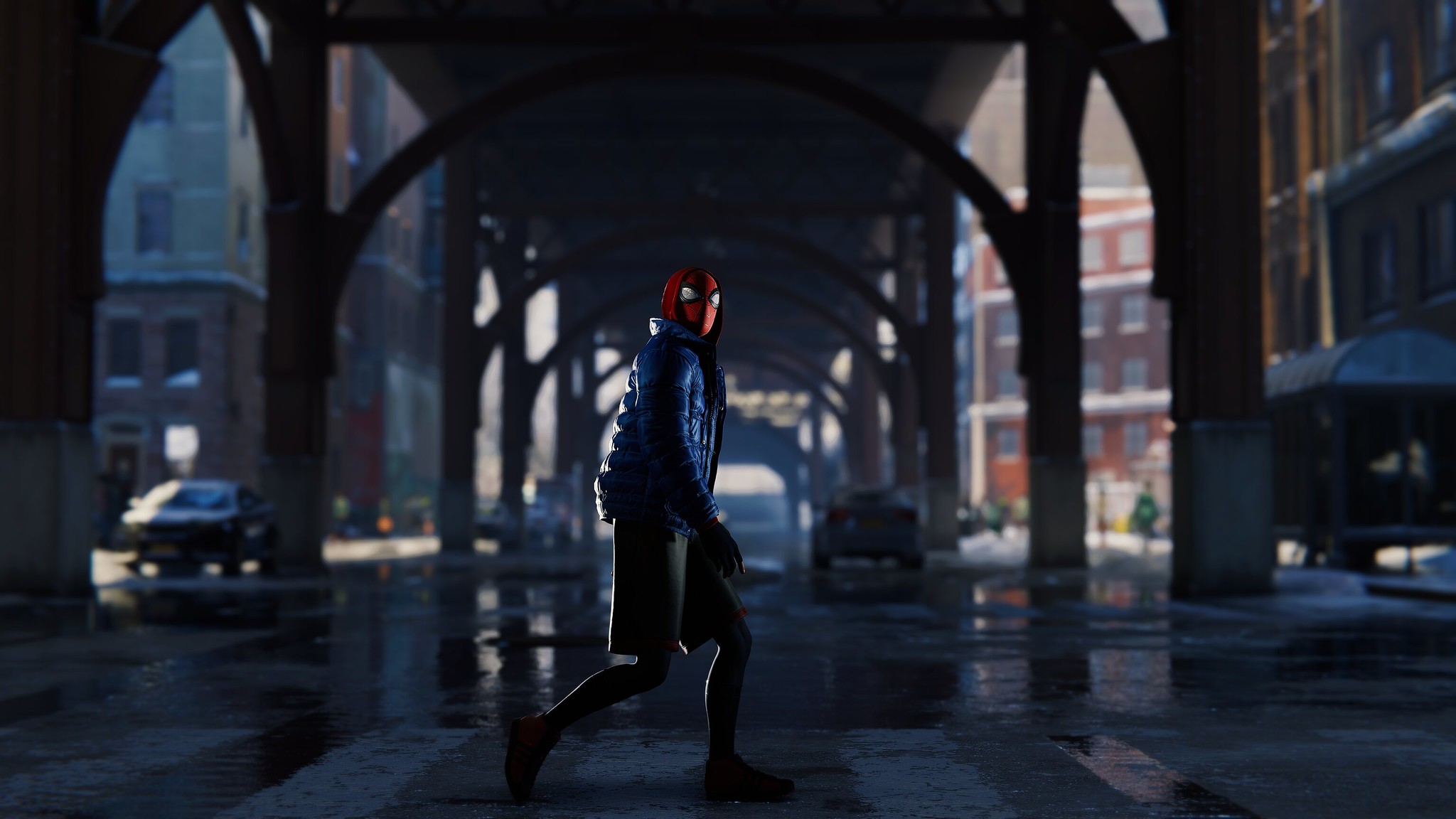In this color, horizontally-oriented photo, a man, dressed in long black shorts, black leggings, black shoes, and a blue puffer jacket, is seen casually walking through a crosswalk under a series of large, dark arches of what appears to be an elevated train structure or freeway overpass. The arches are substantial enough to fit two or three rows of vehicles, and the scene suggests it might have recently rained as the streets glisten with wetness. The man is distinctively wearing a red Spider-Man mask, complete with white and black eyes, partially concealed by a red hood. On the right side, a brick building with a bus stop and awning is visible, while on the left, additional buildings and several vehicles can be seen. The setting is outdoors, during daytime, and although the area under the structure is slightly darker, the cityscape beyond is clearly discernible. The overall impression is of an ordinary street moment given an extraordinary twist by the man's Spider-Man attire.